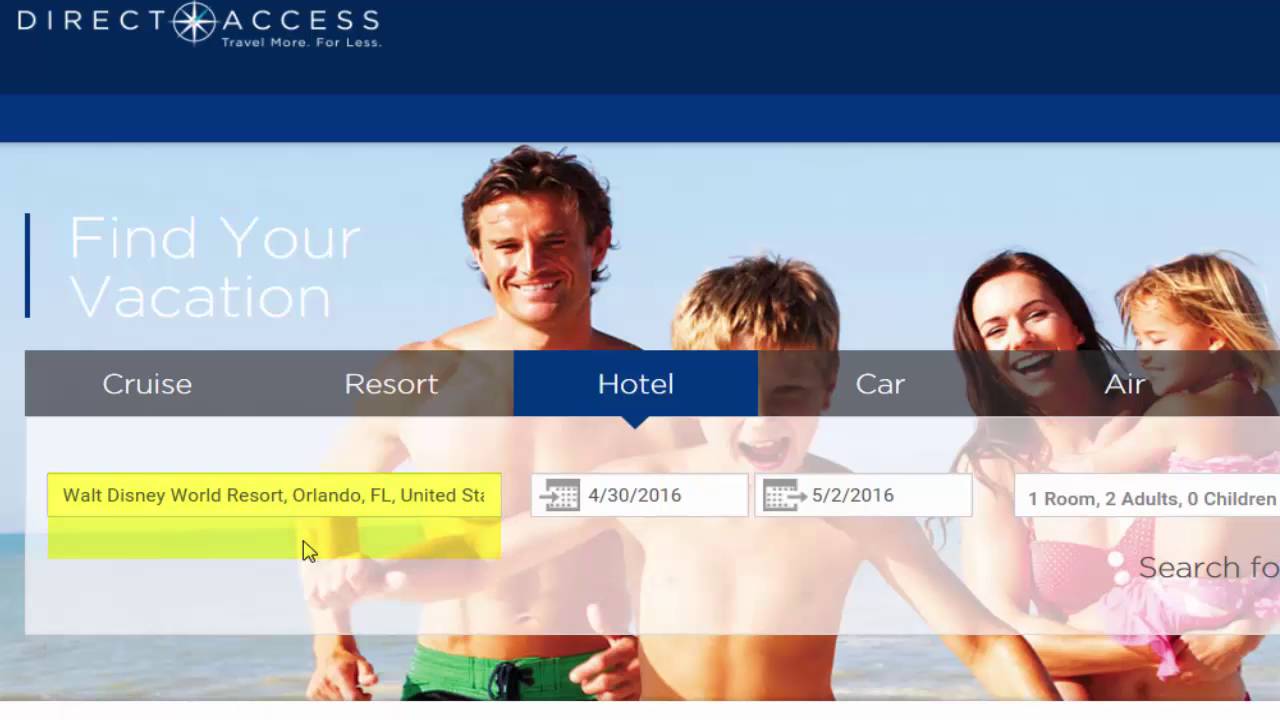In the upper left corner of the image, there's a dark blue banner with the phrase "Travel More for Less." Below it, a lighter blue band transitions into a photo backdrop dominated by a light blue sky. On the left side of the image, the text "Find Your Vacation" is displayed prominently.

A horizontal strip runs across the center of the photograph, listing various travel options: "Cruise," "Resort," "Hotel," "Car," and "Air." Among these options, "Hotel" is highlighted in blue while the others remain gray. Below this strip, there's a highlighted yellow data bar displaying "Walt Disney World Resort, Orlando, Florida, United States," along with details such as "Hotel," dates "4/30/2016 - 5/2/2016," "One Room," "Two Adults," and "Zero Children." A "Search" button is situated within this section, featuring a white, semi-transparent background that allows the underlying photo to be visible.

The backdrop photo captures a joyful family scene: a man and a boy, both shirtless, running ahead; the boy is in front. A woman in a bikini is carrying a girl, who is also wearing a bikini. The beach scene extends downward to reveal a hint of water at the bottom of the image.